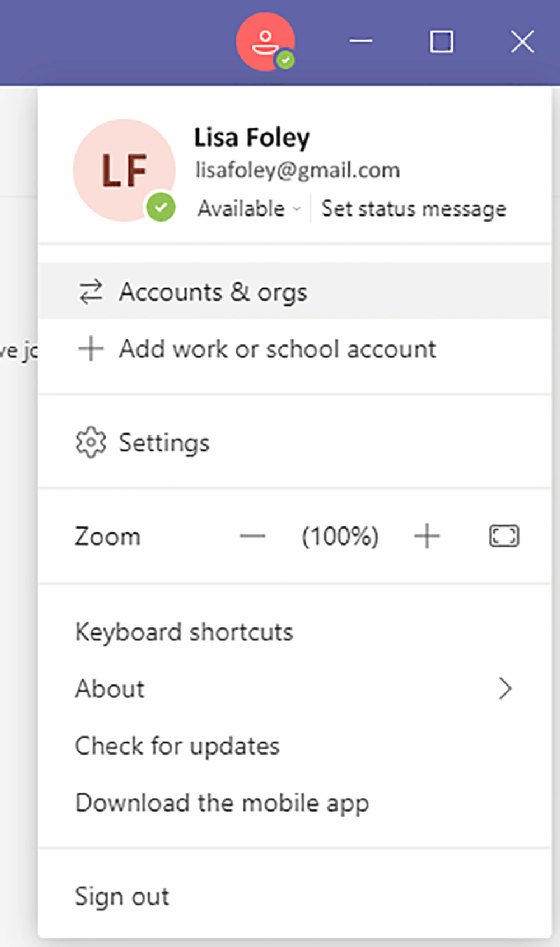Here is the cleaned-up and detailed caption for the image described:

---

The image features a user interface layout. At the very top, there is a white rectangle. Within this white rectangle, a blue rectangle is positioned at the very top, containing several elements. On the right corner of the blue rectangle, there is an 'X' icon. In the center, there is a red circle with a white symbol inside, and next to it, a blue circle filled with green containing a white check mark.

Below these circles, the name "Lisa Foley" is displayed, followed by the email address "LisaFoley@gmail.com." On the left side of this name and email combination, there is a pink circle with the black capital letters ‘L’ and ‘F.’ Adjacent to this, there's a green circle also with a white check mark, and the status "Available" with an option to set a status message.

Further down, the interface lists various sections, sequentially starting with "Accounts and Orgs," alongside an arrow pointing to the right and a subsequent arrow pointing to the left underneath it. Below this section, there is a plus sign with the text "Add work or school account," followed by a settings icon labeled "Settings."

Following this, the word "Zoom" is displayed, flanked by a minus sign on the left and a plus sign on the right of the number "100%," indicating the zoom level of the interface.

Finally, the lower section includes a list of additional options: "Keyboard Shortcuts," "About," "Check for Updates," "Download the Mobile App," and "Sign Out."